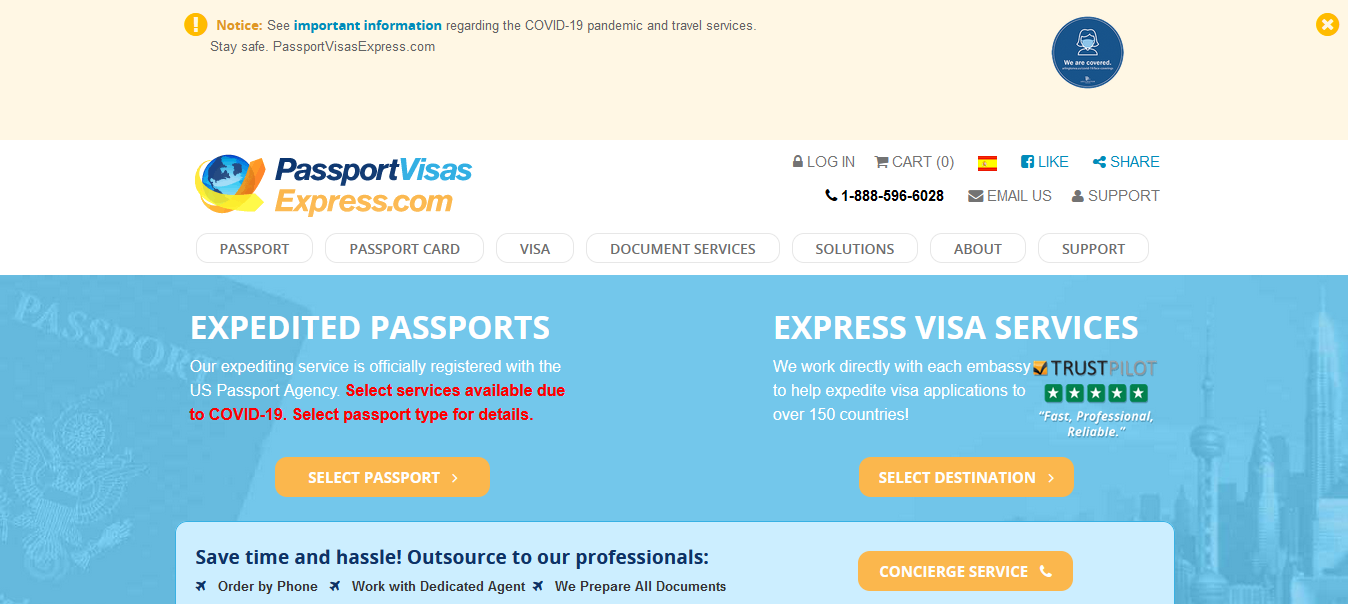The image displays the homepage of PassportVisasExpress.com, featuring a prominent peach-colored header. The header contains an orange attention circle icon alongside a blue image of a person wearing a mask, emphasizing a notice about important COVID-19-related information and travel services.

Centered within the main body of the website, there's a headline stating, "Expedited Passports and Express Visa Services." It highlights that their expediting services are officially registered with the U.S. Passport Agency and mentions the limited availability of select services due to the COVID-19 pandemic. Users are prompted to select their passport type via an orange bar, which initiates the subsequent steps for passport acquisition.

The section below focuses on "Express Visa Services," indicating the company's collaboration with various embassies to expedite visa applications for more than 150 countries. Users can select their destination for specific details.

Additionally, the page features a Trustpilot insignia, underscored with the words "fast, professional, reliable." A section beneath this encourages users to "save time and hassle" by outsourcing their needs to the company's professionals, with an option to click for concierge service assistance.